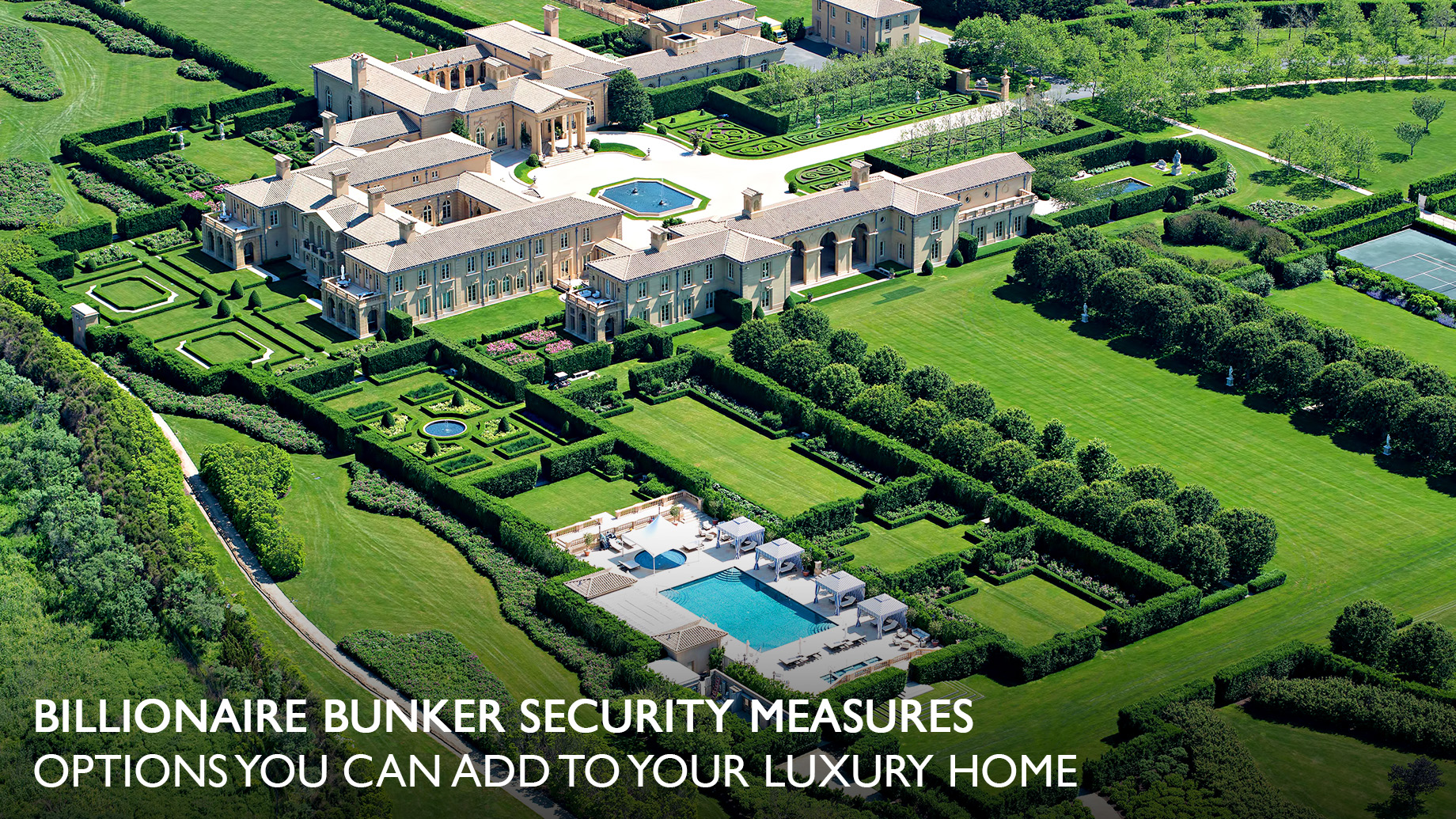This detailed aerial photograph captures a sprawling, luxurious estate, known as a "billionaire bunker," with various security measures and opulent features. Dominating the image is a large, beige mansion with three main wings, adorned with multiple white windows and Roman columns, exuding grandeur and elegance. Surrounding the mansion is an expertly manicured landscape, showcasing lush green lawns, well-tended trees, and hedges. 

Prominently featured in the foreground is a grand swimming pool, accompanied by several tables and enclosed by pristine hedges. Notably, the estate boasts a second pool, emphasizing its luxurious appeal. A long driveway encircles a central fountain, connecting the mansion's sections and enhancing the estate's majestic ambiance.

Towards the top center, various auxiliary buildings, including a guest house, complement the main residence. In the far right of the image, a tennis court is visible, tucked behind strategically placed bushes, adding to the recreational allure of the property.

The caption in the bottom left corner reads, "billionaire bunker security measures options you can add to your luxury home," underlining the exclusivity and high-level security features of this immense, meticulously maintained estate.